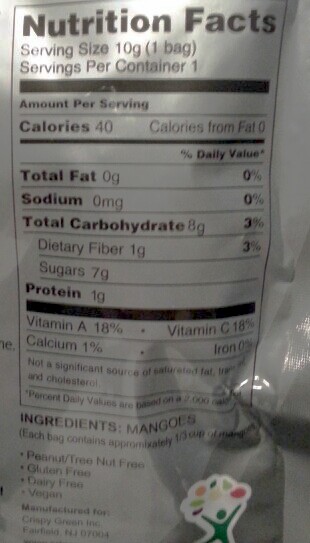The image displays a detailed nutrition label for a snack product. The label is titled "Nutrition Facts" and indicates a serving size of 10 grams (1 bag), with one serving per container. The nutritional breakdown per serving includes 40 calories, with 0 calories from fat. The label further details the contents as follows: 

- Total Fat: 0g
- Sodium: [Amount not specified]
- Total Carbohydrates: [Amount not specified]
  - Dietary Fiber: [Amount not specified]
  - Sugars: [Amount not specified]
- Protein: [Amount not specified]

The label also highlights specific daily values of various nutrients based on a 2,000 calorie diet:

- Vitamin A: 18%
- Vitamin C: 18%
- Calcium: 1%
- Iron: 0%

Additionally, the label notes that the product contains mangoes as its ingredient, with each bag equivalent to approximately one-third of a cup. The product boasts several dietary accommodations, being peanut-free, nut-free, gluten-free, dairy-free, and vegan.

The label states that the product is manufactured for Crispy Green Inc. in Fairfield, New Jersey. At the bottom of the label, there is a colorful sticker depicting a person holding a variety of fruits, contributing to the overall healthy and vibrant presentation of the product.